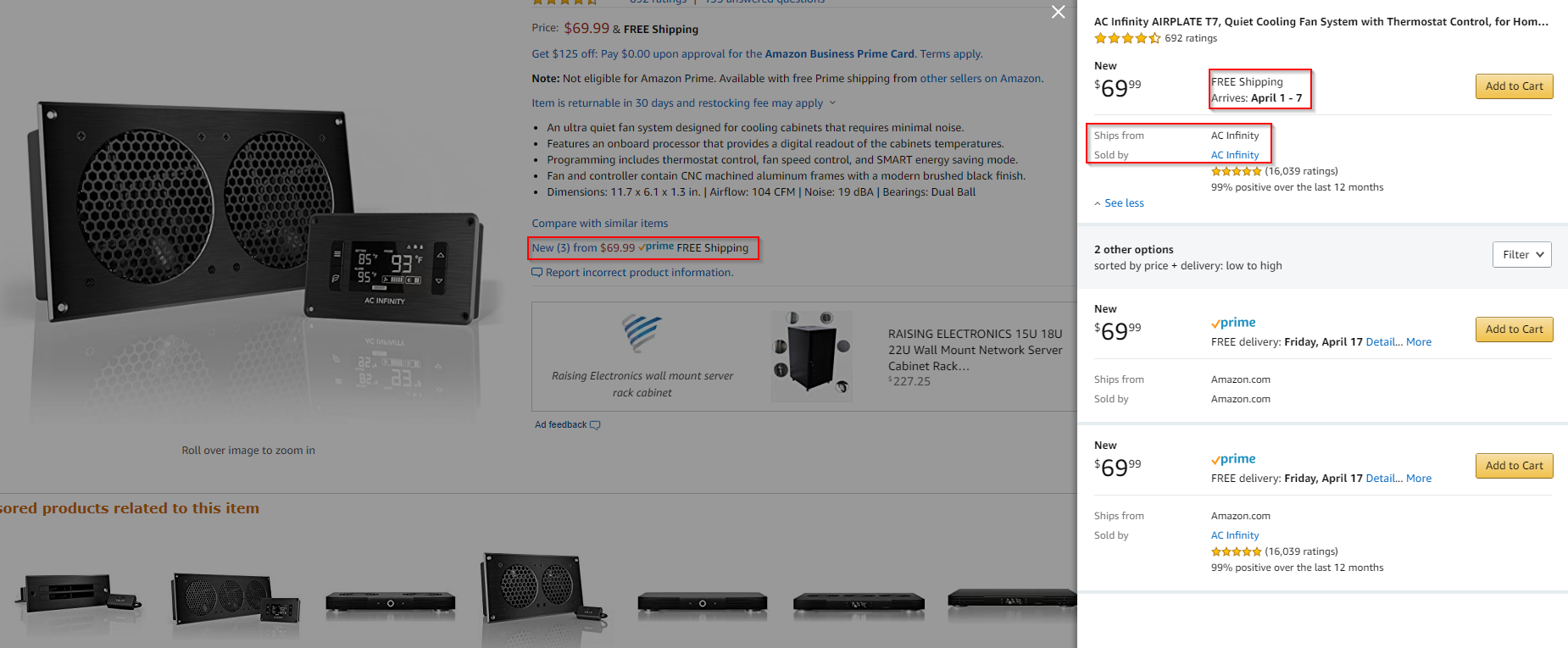The image displays an Amazon listing featuring an audio receiver and speaker set. On the left side of the page, there is a product image of the black receiver with white text on its display, accompanied by matching speakers. These items are presented against a white background. Below the main image, several additional pictures of the product are displayed.

In the upper right corner of the page, the price is prominently shown as $69.99, with a note indicating free shipping. The shipping details mention a delivery window between April 1st and April 7th. Both the price and shipping information are enclosed in red boxes, emphasizing their importance.

To the right, there are options to purchase, including an "Add to Cart" button highlighted in yellow with black text. The "Ship from and sold by" information is also highlighted in a red box, adding further clarity for potential buyers.